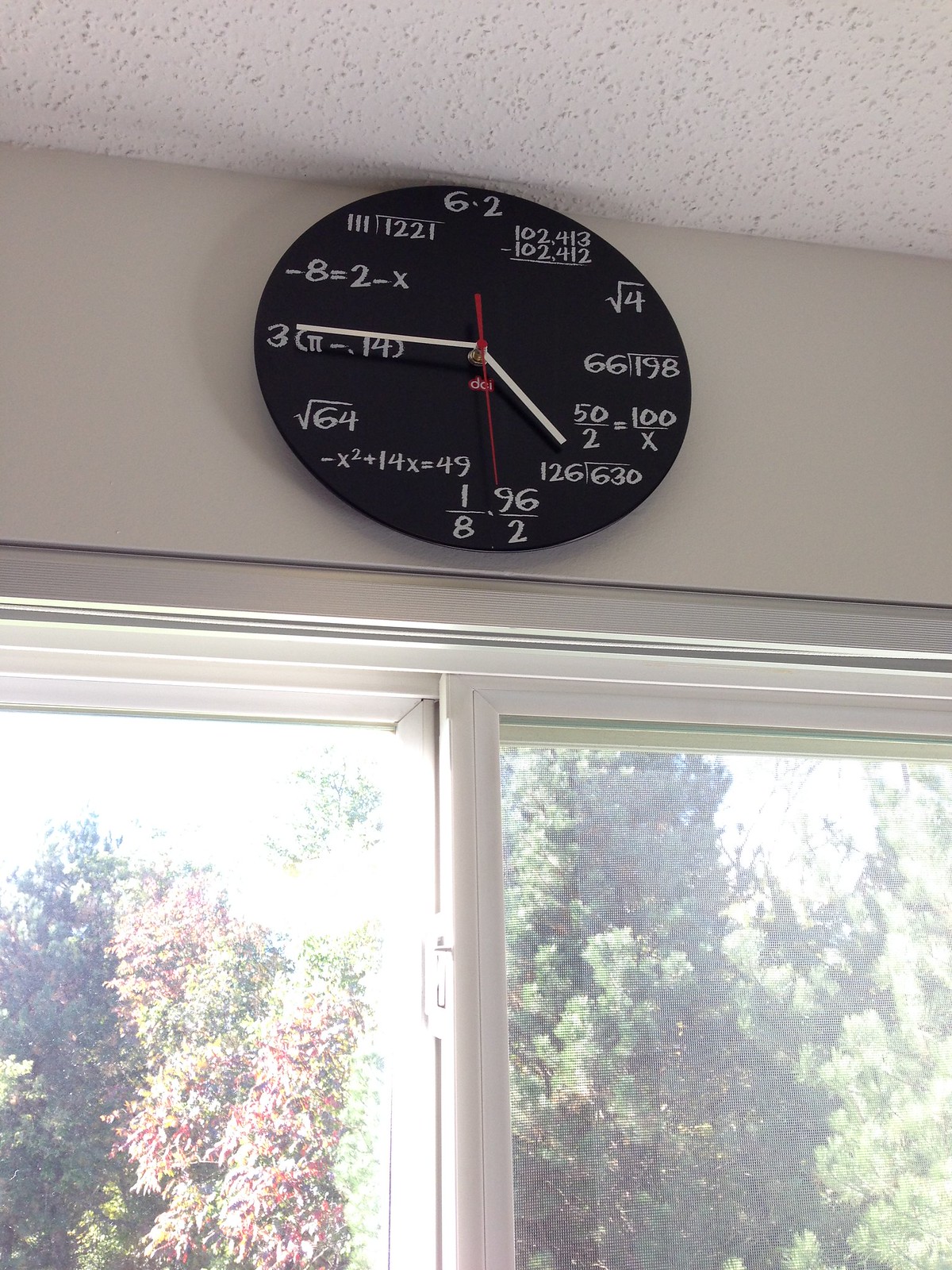A photograph features a unique clock mounted above a window. The clock, with a black face, showcases white minute and hour hands, along with a red second hand. Instead of traditional numbers, the clock face is adorned with various mathematical formulas, such as 6x2 representing 12 and √4 representing 2. The text on the clock has a chalkboard-style aesthetic. The clock is set against a white wall, and above it, a textured white drop ceiling is visible. Below the clock, a window with a white frame provides a view of the outside, where trees adorned with mostly green and some red foliage can be seen. The scene is captured during daytime, adding a bright and airy feel to the image.